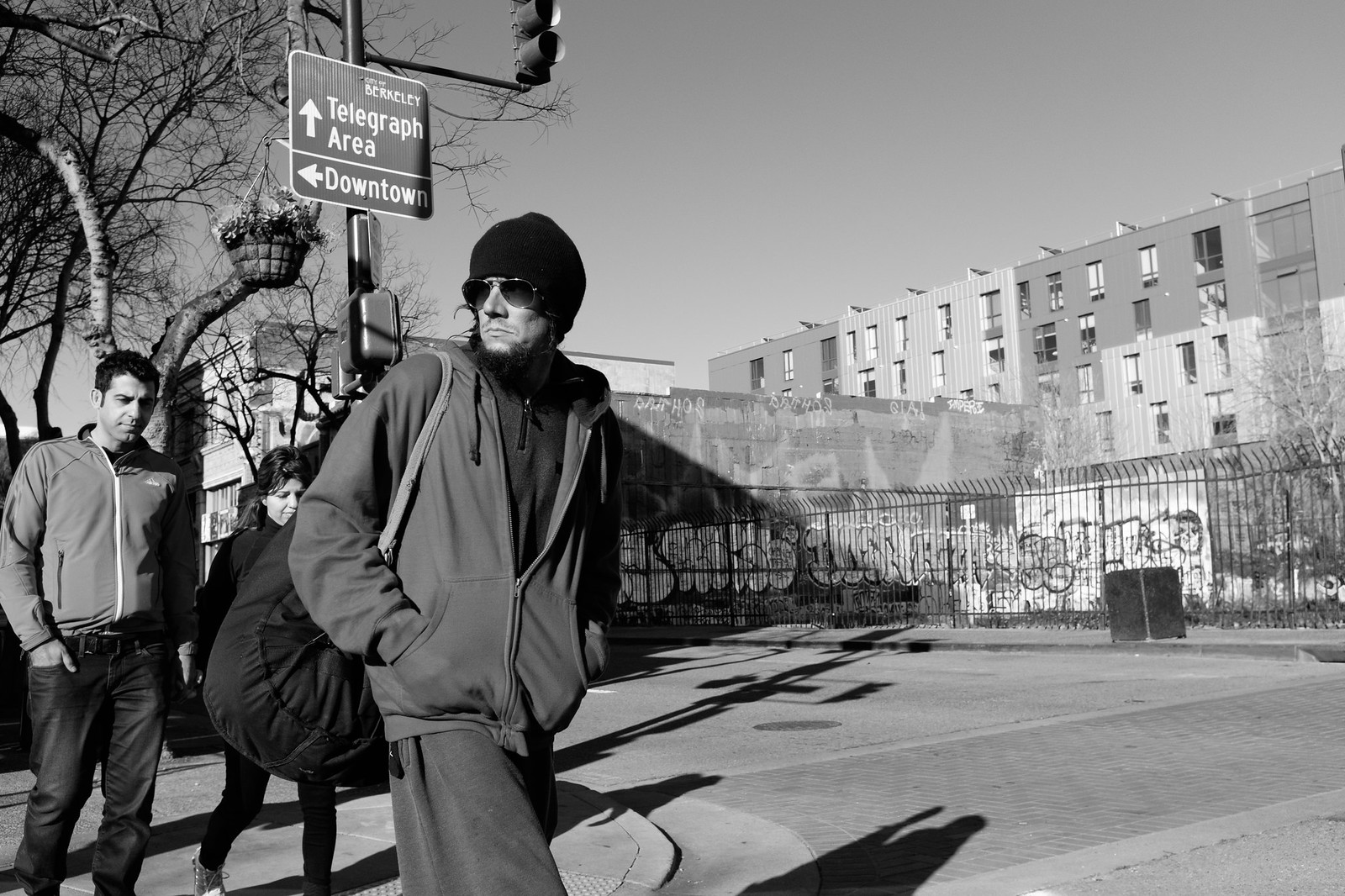This professionally shot black and white photograph captures a dynamic street scene at an intersection, likely located in Berkeley, as indicated by the signs in the image. On the left side of the frame, a man stands prominently. He is wearing a partially zipped hooded sweatshirt, a black beanie, sunglasses, and has his hands in his pockets. Additionally, he carries a bag over his right shoulder and has a somewhat stern demeanor. Behind him, a couple walks closely together, possibly holding hands. The man in the couple wears a lighter hooded jacket, while the woman wears a long black coat.

The intersection is paved with what appears to be brick or cobblestone, adding texture to the street scene. On the right side of the image, a cluster of older, possibly dilapidated buildings and apartments stands behind a metal fence adorned with graffiti. A sidewalk runs in front of this fence, and a garbage can is visible nearby. Trees provide some greenery, and a hanging basket can be seen above the people.

A stoplight with directional signs hangs above the street, indicating "Telegraph Area" with an arrow pointing upwards and "Downtown" with an arrow pointing to the left. These details contribute to the urban atmosphere of the scene. The overall composition of the photograph, framed in a horizontal rectangular format, creates a vivid and detailed snapshot of urban life during what appears to be a daytime moment.